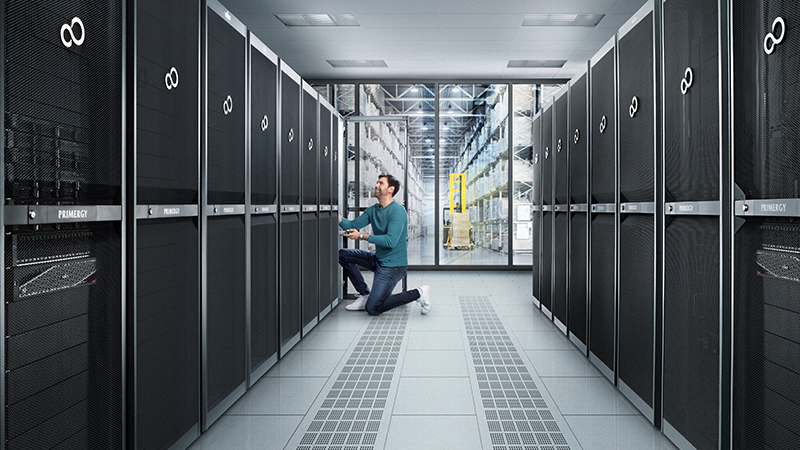This image captures a man in a futuristic, sleek server room, donned in a turquoise long-sleeve shirt, blue jeans, and white shoes. He's kneeling in front of a black server cabinet on the left side, smiling and appearing engaged in his work. The server room is compact yet modern, with about 8-10 black server cabinets on each side, all closed so the inner components aren't visible. The floor is white with gray ventilated grates running along the sides. Behind the man, through large glass windows, lies a spacious, tall warehouse with rows of shelves stacked high with white packages. Prominently, a yellow forklift is in sight, carrying brown boxes, indicative of the warehouse's bustling activity. The entire scene strikes a balance between high-tech infrastructure and industrious warehouse operations, underscored by the clean, organized aesthetic of both the server room and the warehouse beyond.